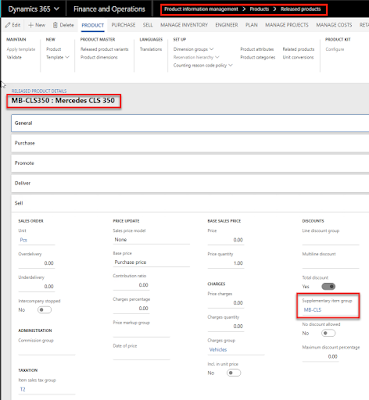### Descriptive Caption for an Image of the Dynamics 365 Page

This image is a screenshot of a Dynamics 365 interface, specifically, the "Finance and Operations" section tailored for a car dealership. The navigation menu at the top features options such as "Product Information Management," "Products," and "Retired Products" highlighted within a red box. 

Beneath the main navigation, a secondary menu includes several functional categories: "File New Device Product," "Purchase," "Sell," "Manage Inventory," "Engineer," "Plan," "Manage Projects," and "Manage Costs." However, due to the image size, the text in this area is challenging to read clearly.

Continuing further down, there is a section that mentions "MB-CLS350 Mercedes CLS350," indicating the car model being managed or sold. Above this, a blue hyperlink labeled "Related Product Details" is visible, with a highlighted orange or red box around the Mercedes option.

Below, there are tabs labeled "General," "Purchase," "Favorite," "Deliver," and "Sell," with the "Sell" tab currently active, displaying various sales-related options. Towards the bottom right, approximately 20% up from the lower edge, there is another red box, though the contents within it cannot be deciphered due to the image's small size.